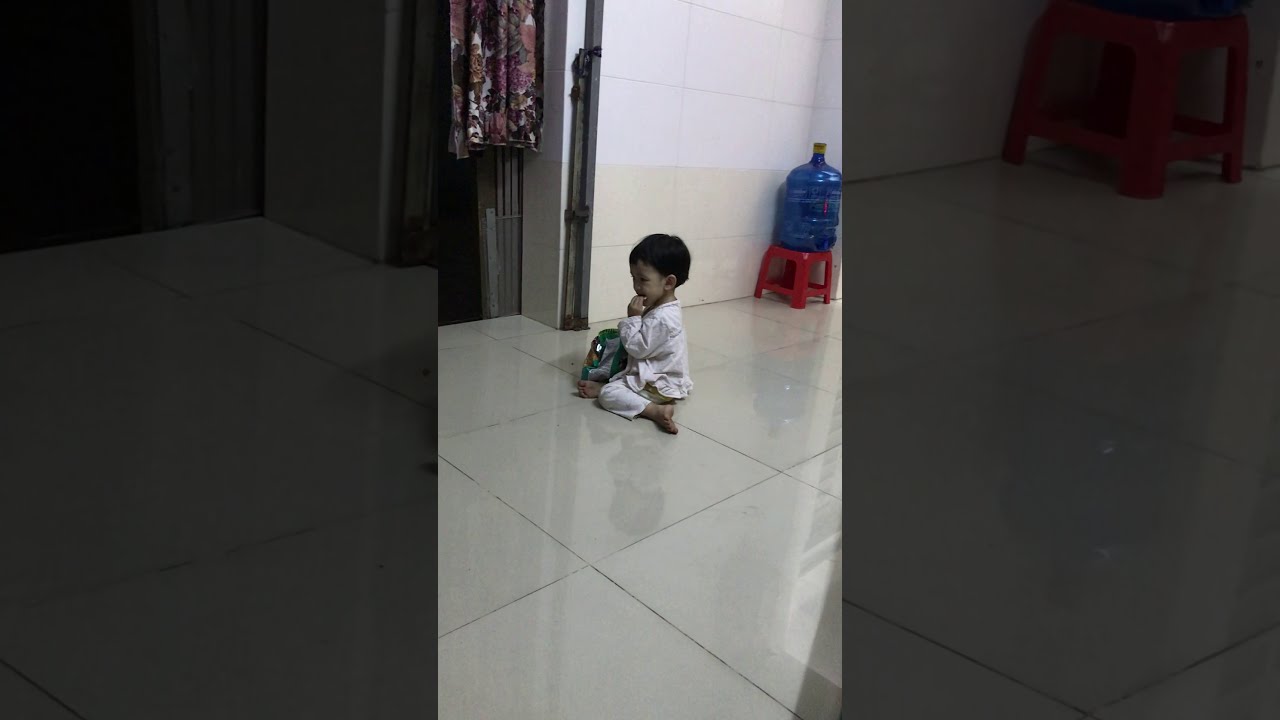In the image, a young toddler with dark black, short hair and brownish skin is sitting on large, shiny, square tiled flooring, likely in a kitchen. The child, dressed in a white long-sleeved shirt and white pants, is barefoot and holds a green plastic bag from which they are eating a snack. The room features tannish and white tiled walls. To the left, there is an open doorway with a flower-patterned curtain. In the right corner of the room, a small red stool supports a large water jug, which appears to be in use, possibly for collecting coins. The black framing on the sides suggests a simple, focused photograph emphasizing the toddler in their pajamas, engaging with the green bag of snacks.